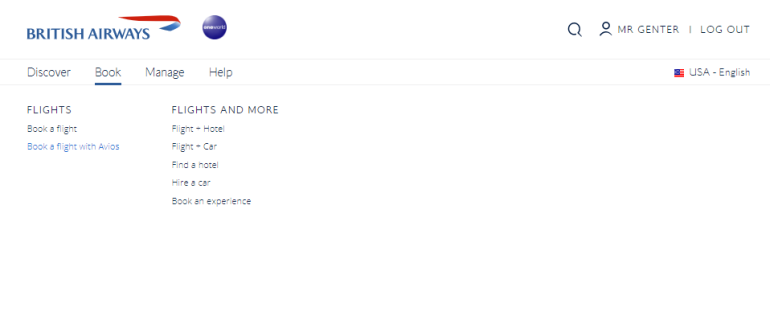Screenshot of the British Airways Website:

At the very top of the screen, the British Airways logo is prominently displayed on the far left, alongside the One World Airline Alliance emblem, indicating the airline's membership in the alliance. On the upper-right corner, there's an hourglass icon for accessing the search function, next to a personal icon labeled "Mr. Jenter," suggesting that Mr. Jenter is currently logged into his British Airways account. This section also features a "Log out" option, allowing Mr. Jenter to exit his account.

Beneath the logo bar, a navigation menu spans the width of the screen with the options: Discover, Book, Manage, Help, and USA English, offering language and region customization. The "Book" tab is selected in this screenshot, revealing a submenu with various booking options. Users can choose to book a flight directly or with Avios points, and explore further travel arrangements such as flight + hotel, flight + car, finding a hotel, hiring a car, or booking an experience. This submenu serves as a gateway to the British Airways travel portal, providing comprehensive options for planning an entire journey beyond just flights.